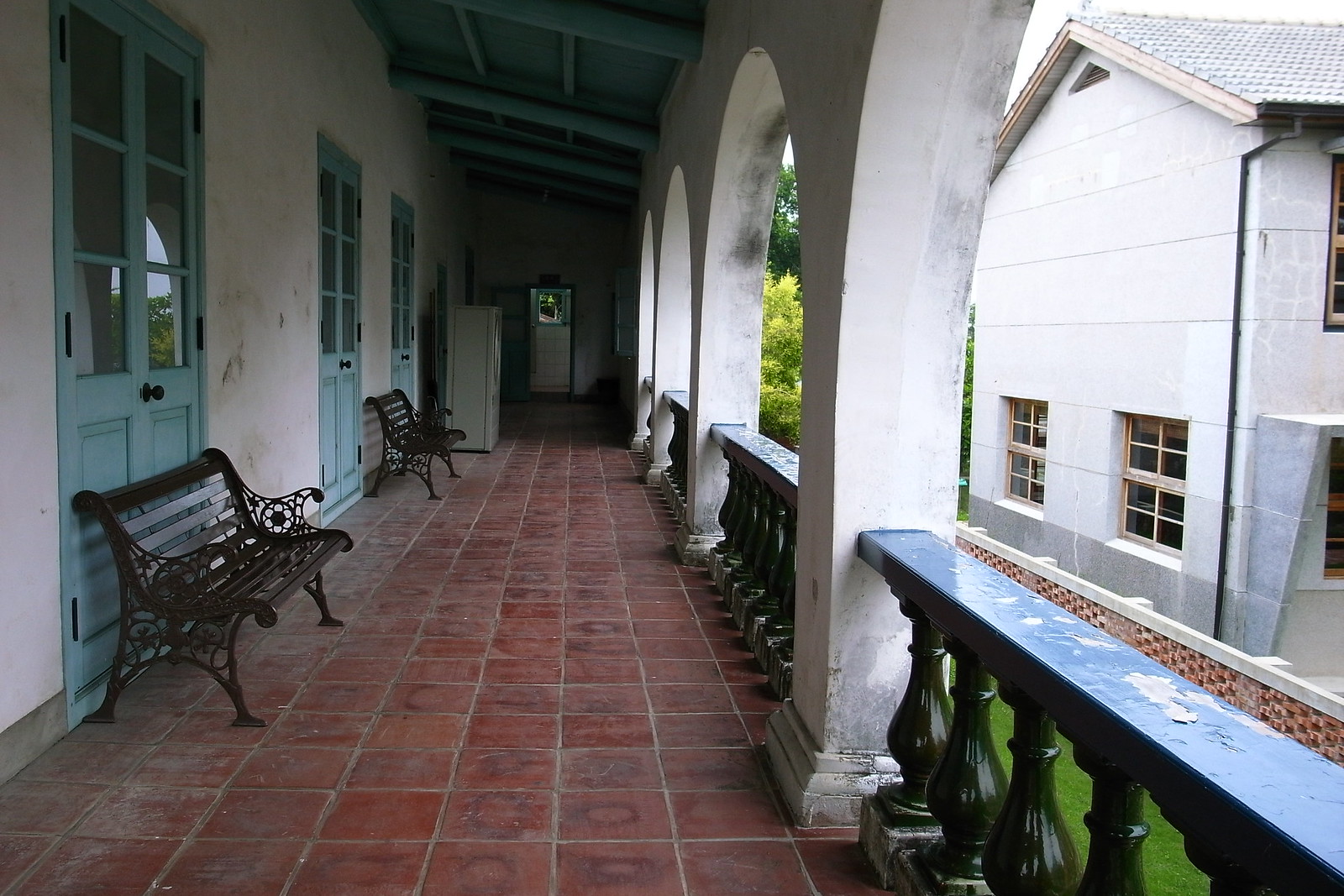The image shows a veranda on the upper floor of a Spanish-style building, reminiscent of a lanai or elongated balcony. The floor is laid in dark reddish-brown tiles with light brown grout, giving it a distinctive look. On the right side, ornate wooden railings, possibly dark green, feature vase-shaped posts topped by a horizontal bar, creating a series of archways supported by white rectangular columns. The railings and archways have peeling black paint in some areas, adding a weathered charm. Through these archways, we glimpse a neatly manicured grassy area and a neighboring building with a brick wall.

To the left of the image, the building’s exterior wall is white, adorned with a series of three sets of light blue double doors featuring windows at the top. Two wrought iron and wooden benches are strategically placed in front of these doors, providing seating options. In the background, a white refrigerator is partially visible against the wall. The veranda’s ceiling, angled and blue, provides a contrasting overhead structure. Overall, the detailed scene captures an inviting upper-level walkway, blending architectural details and casual elements with a view of the adjacent building's white facade and gray roof.